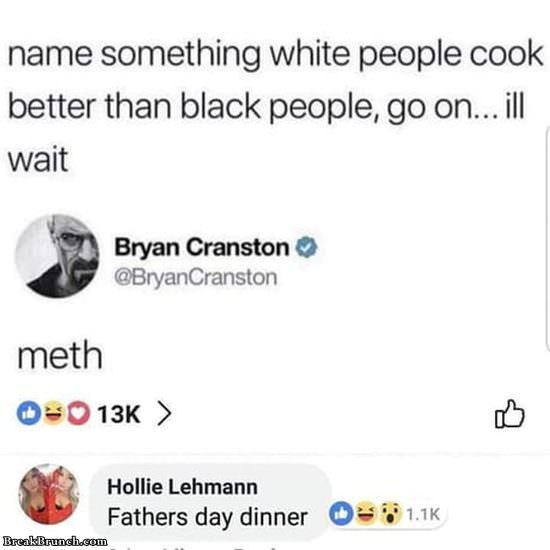This is a detailed screenshot from Twitter, displaying a humorous interaction initiated by a user and responded to by actor Bryan Cranston. The verified account, denoted by a blue checkmark next to the username @BryanCranston, features an avatar representing his iconic character from "Breaking Bad," a white man with glasses, a goatee, and a mustache.

Above Bryan Cranston's tweet, a provocative question was posted: "Name something white people cook better than Black people. Go on, I'll wait." In response, Cranston humorously replied, "Meth." This tweet has garnered significant engagement, illustrated by icons and figures below it: a blue circle encapsulating a thumbs-up icon, a laughing smiley emoji, and a heart emoji against a pink background, accompanied by the number "13K." Additionally, a thumbs-up icon without a circle appears on the far right of the same row.

Following Cranston's popular tweet, Holly Lemon, a presumably young blonde woman, judging by her dual-faced avatar, chimed in with her response, "Father's Day dinner." Her reply has further elicited interactions signified by a blue circle thumbs-up, two smiley emojis, and "1.1K" next to it.